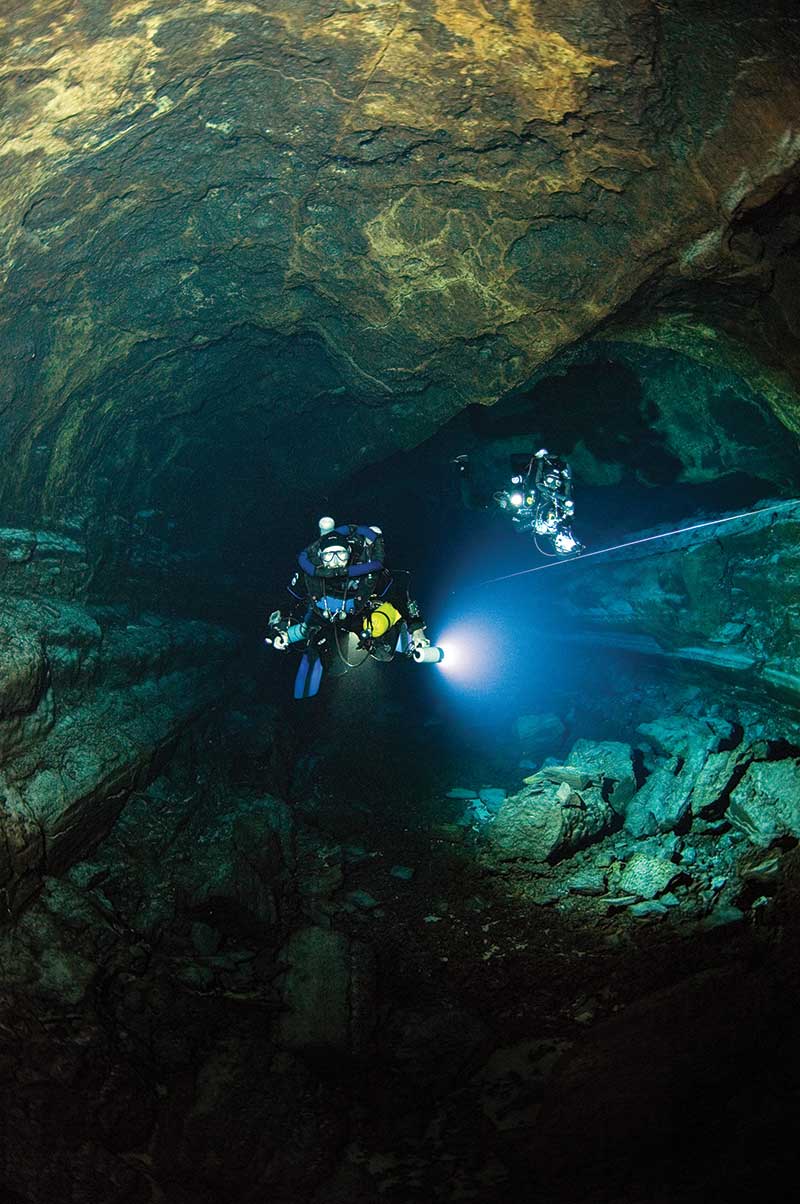This captivating underwater image depicts two scuba divers exploring a vast and shadowy cave. Both divers, clad in purple and black suits with full scuba gear, including large breathing apparatuses and oxygen tanks, are centrally positioned and equipped with flashlights that pierce the pitch-black surroundings. The illumination from their gear reveals jagged cave walls and a rocky floor scattered with various debris on the bottom right. A white guide line runs alongside the right side of the image, assisting the divers' navigation through the cavernous, tubular passage. The atmosphere feels thrilling and mysterious, encapsulating the sense of adventure and exploration.